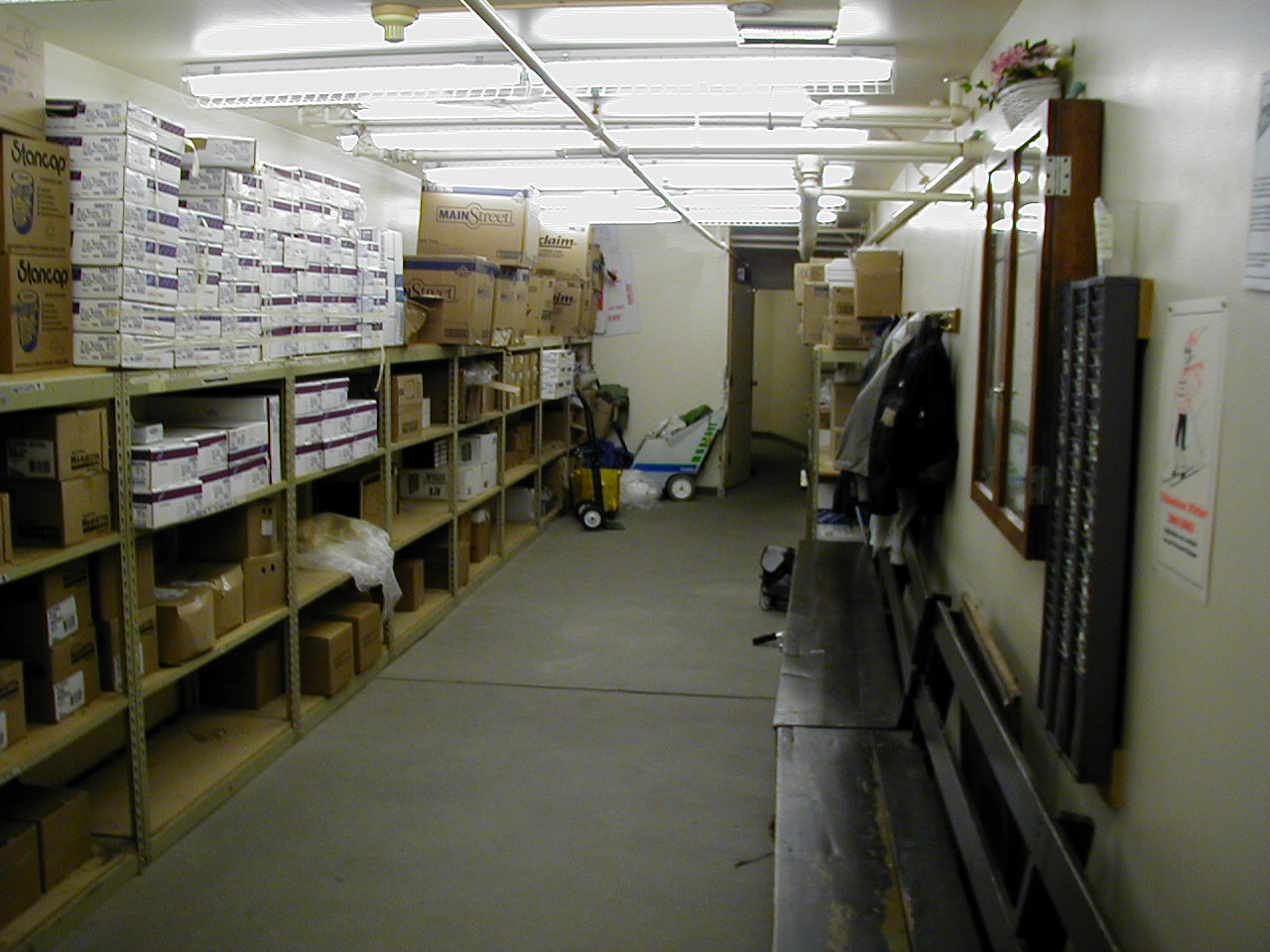The image depicts an indoor photograph of a small warehouse or storeroom featuring a wide aisle with a gray concrete floor. Along the right wall, which is painted white, there are two elongated black wooden benches, possibly used for sitting to put on or remove shoes or skates. Above these benches, there are coat hooks with various coats hanging, and a display case containing a potted plant. Also visible is a rack holding time cards, indicating a possible employee area. The storeroom is brightly lit by linear fluorescent lights attached to the white ceiling. The left wall is lined with metal shelving units holding numerous brown and white cardboard boxes, including ones labeled "Main Street" and "STANCAP.” Additional utility items such as truck carts used for hauling heavy objects and a floor washer or waxer are also discernible. A picture of a skier decorates the wall, providing a touch of personality to the industrial space. Various pipes and a smoke detector are seen on the ceiling, indicative of the room’s functional design. At the far end of the aisle, an open doorway leads to another section of the storeroom.